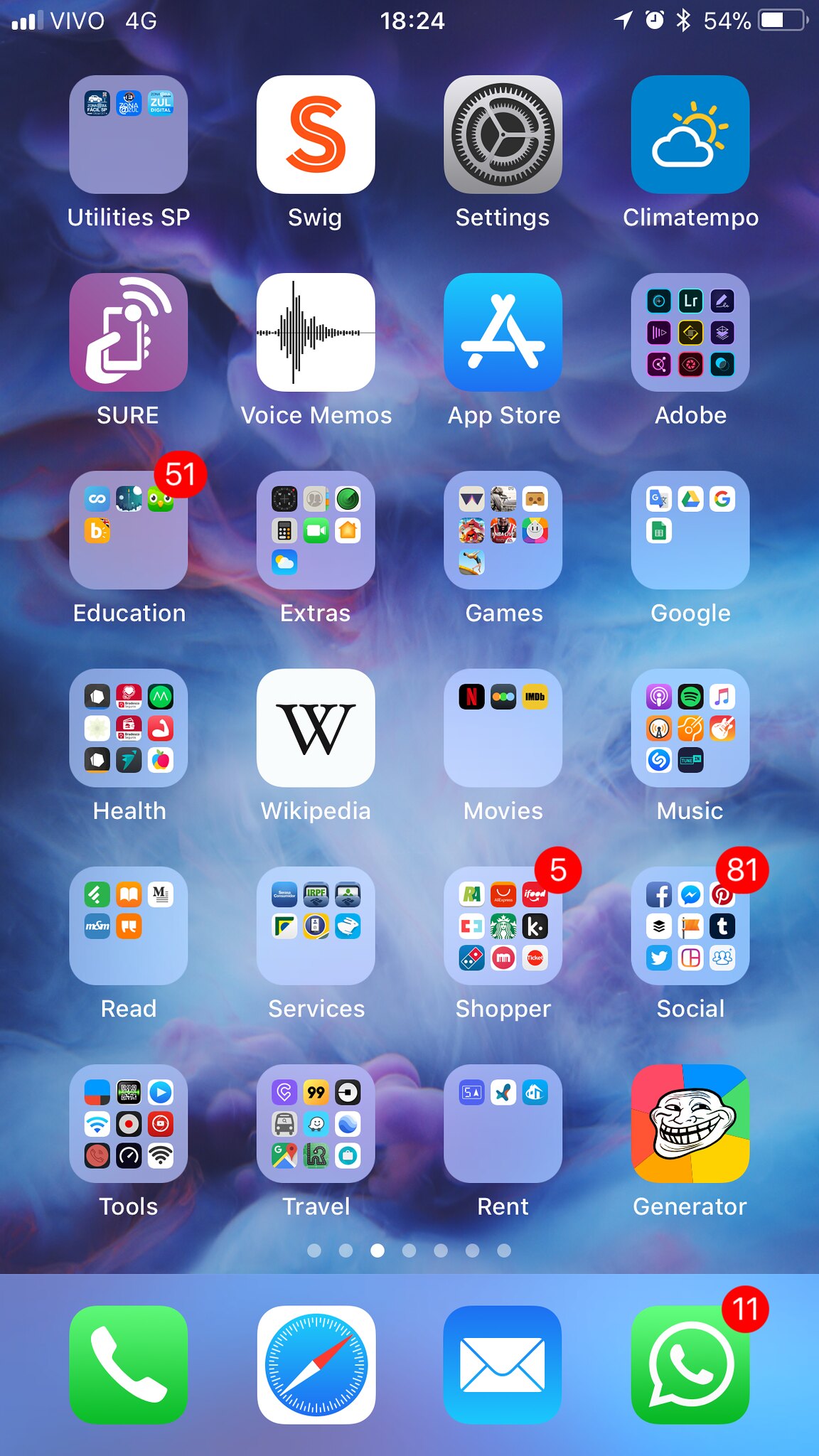Screenshot of an iPhone Home Screen

This image captures a detailed view of an iPhone's home screen, though the specific model is not identifiable. The background wallpaper features an intricate pattern of swirling purple and blue smoke, lending a visually pleasing backdrop to the array of apps. 

Prominently displayed in the bottom dock, which remains constant across all app pages, are four essential apps: Phone, Safari, Mail, and WhatsApp. At the bottom of the screen, there are seven dots indicating a total of seven available pages filled with various apps.

On the home screen, there are a multitude of apps and organized app groups. Some of the individual apps visible include Swig, Settings, ClimaTempo, App Store, Voice Memos, Shore, Wikipedia, and Generator. 

In addition to individual apps, there are numerous folders categorizing apps under specific utilities such as Adobe, Games, Google Extras, Education, Health, Movies, Music, Services, Shopper, Social, Travel, Tools, Rent, and Read. The presence of these folders indicates a well-organized and diverse range of applications.

At the top of the screen, the status bar shows that the user is connected via Vivo 4G network. The current time displayed is 18:24, and the battery level is at 54%.